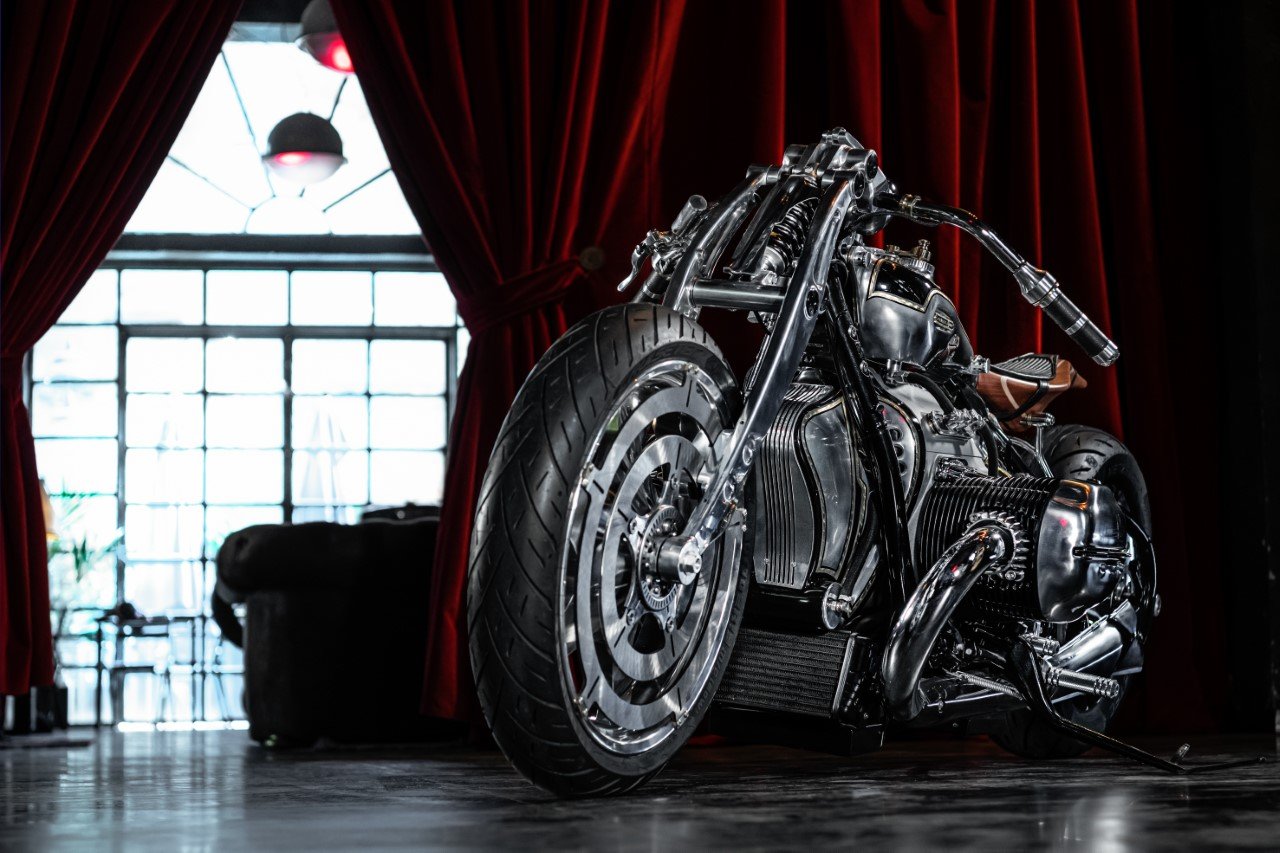The image showcases a chromed-out motorcycle prominently displayed inside a room with red velvet curtains. The motorcycle, angled diagonally, has its front left side closer to the camera while the back tire, partially visible, is farther to the right. The motorcycle features black-bordered chrome components, with particularly narrow black front tires with silver spokes. The reflective floor under the motorcycle is gray and black.

In the background, a large red curtain spans from the right to two-thirds across the screen and is partially parted to the left, revealing a seating area with a couch, a table, and windows and doors made of clear glass. The room is well-lit with ceiling lights that have white covers emitting a red hue. This setup gives the impression of a showroom or dealership, with the sun shining through the glass wall, enhancing the display of the motorcycle.